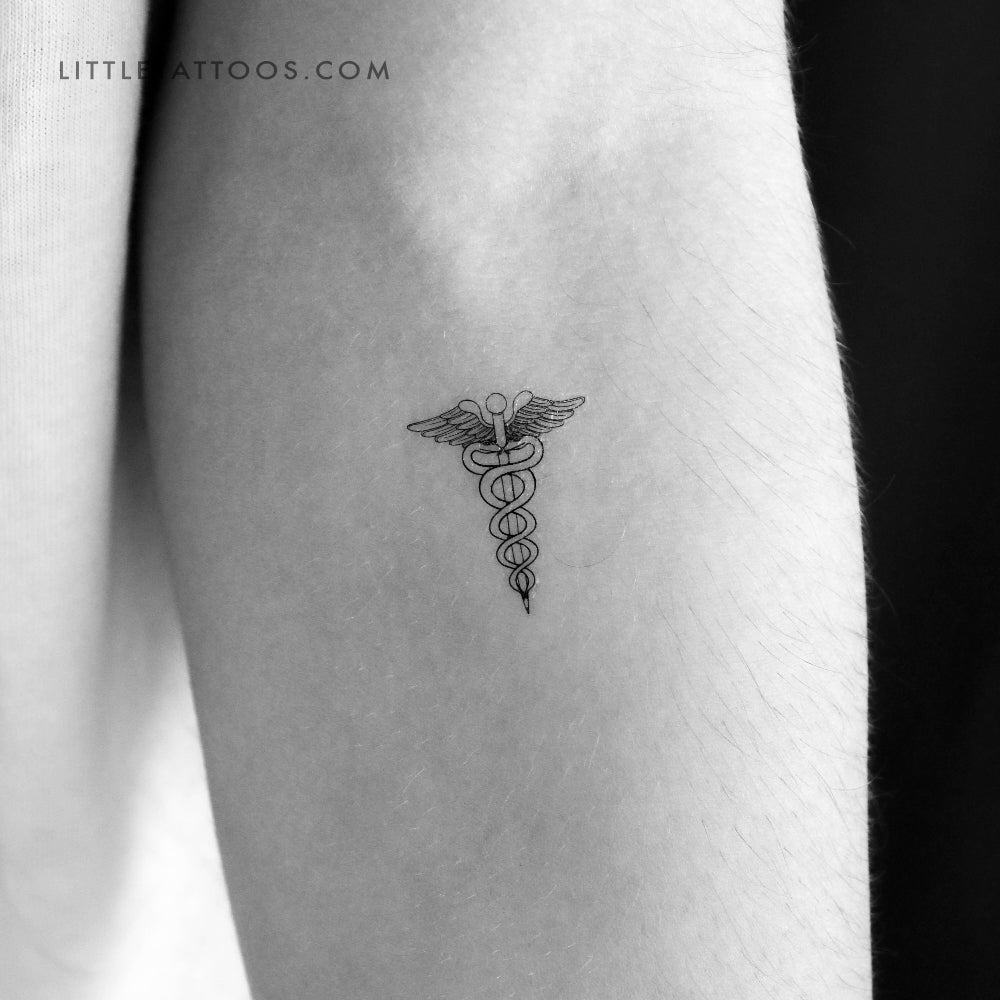The image is a black and white close-up of a small tattoo on the inner forearm near the elbow, with a website watermark "littletattoos.com" in the top left corner. The tattoo, likely about the size of a penny or an inch and a half to two inches in length, depicts a traditional caduceus—a symbol often associated with medicine. This includes a staff entwined by two serpents with wings. The arm appears to be of a light-skinned person with some visible hair, suggesting it might belong to a man. A bit of a t-shirt is visible on the left side, and the background is black, emphasizing the zoomed-in focus on the intricately detailed tattoo.